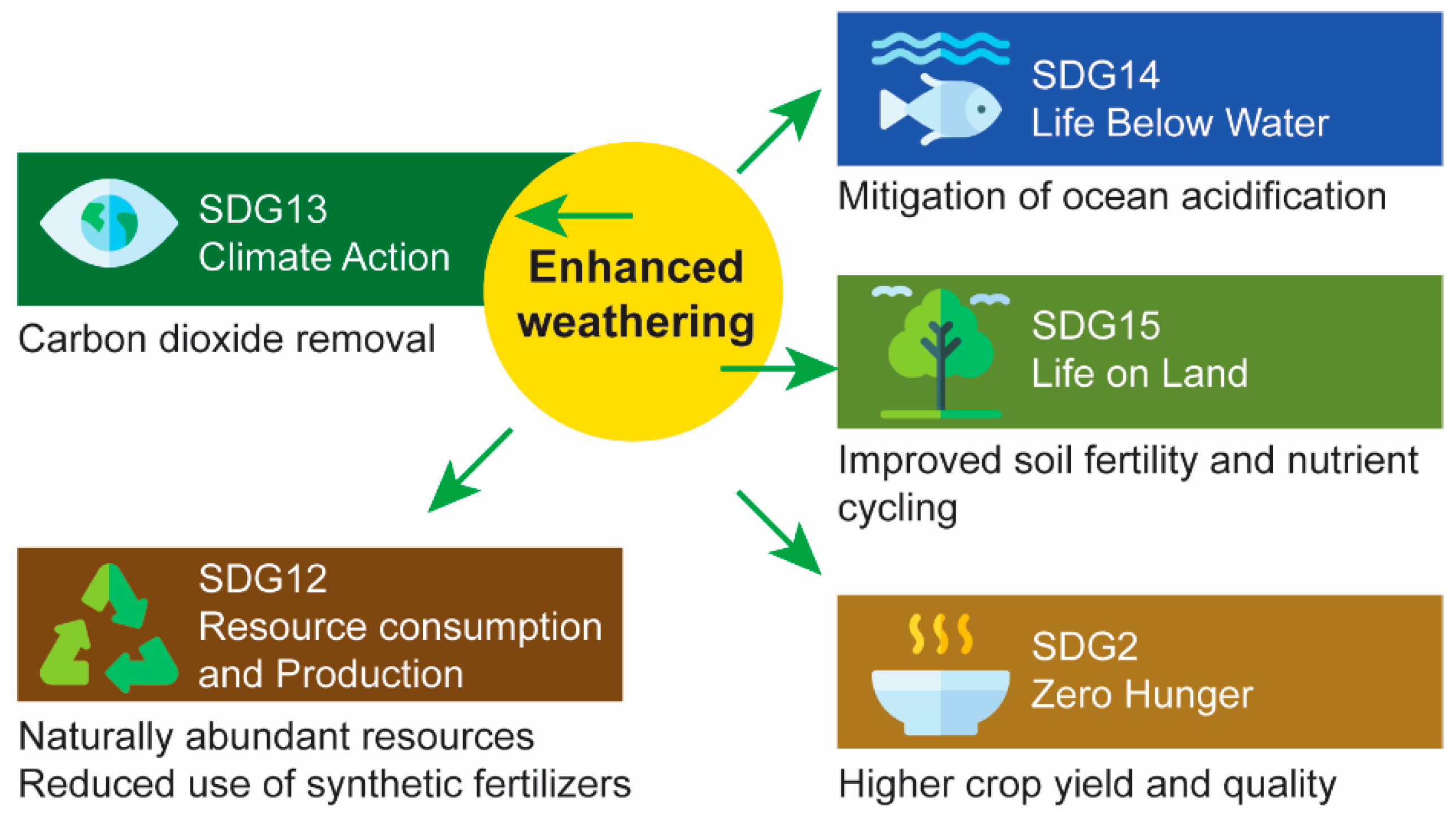The image is a detailed pictogram that illustrates the concept of enhanced weathering and its relevance to various Sustainable Development Goals (SDGs). At the center of the image, a yellow sun encases the main text, "Enhanced Weathering," written in black. Green arrows radiate from this central circle, pointing to different colored banners, each representing a specific SDG and accompanied by corresponding icons and captions.

To the left, a green banner labeled "SDG 13 Climate Action" highlights "Carbon Dioxide Removal." Below it, a brown banner tagged "SDG 12 Resource Consumption and Production" includes a green recycling symbol and mentions "Naturally Abundant Resources" and the "Reduction of Synthetic Fertilizers."

On the right side of the image, another green arrow leads to a blue banner for "SDG 14 Life Below Water," featuring a fish icon and noting the "Mitigation of Ocean Acidification." Below this, a green banner for "SDG 15 Life on Land" shows a tree and bird icon, with the caption "Improved Soil Fertility and Nutrient Cycling." Finally, a light brown banner at the bottom right, labeled "SDG 2 Zero Hunger," includes an image of a steaming bowl and emphasizes "Higher Crop Yield and Quality."

Overall, the pictogram effectively conveys complex scientific information about enhanced weathering and its multifaceted benefits across different SDGs, using distinct colors, icons, and detailed captions.